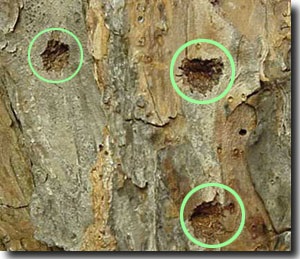This image is a small outdoor photograph, approximately an inch and a half wide and an inch and a quarter high, capturing what appears to be the textured side of a tree trunk. The photograph, showcasing light tan and gray hues, evokes a stone-like appearance but is actually the rugged, flaky bark of a tree. The bark exhibits areas where it is raised and appears ready to peel off. There are three distinct indentations in the bark, highlighted by mint green circles: one in the upper left corner, one at the top center of the right side, and one at the bottom center of the right side. Each indentation suggests damage, possibly from pecking, and the surface is marked by additional minor holes, accentuating its rough texture. The photograph's shadow on a white background suggests it may be mounted or part of a digital artwork.